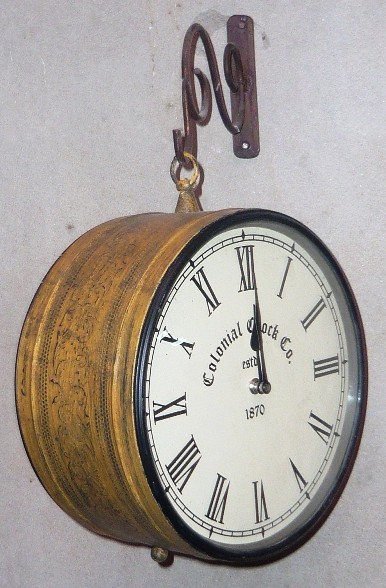Hanging on a rough-hewn stone wall is an antique clock. A sturdy metal hook secures the clock, leading to a prominent ring at the top. The clock itself has a striking brown body adorned with black dots on both its left and right sides. On the right side, the clock face reveals intricate details: at the top, it is inscribed with the words "Colonial Clock Co.," and the center prominently displays the year "1870." The roman numerals marking the hours encircle the face, starting from XII at the top, and sequentially listed as I, II, III, IV, V, VI, VII, VIII, IX, X, XI, and XII again. Encircling the mechanism is a black rim, and the entire face is protected by a covering that appears to be either glass or plastic. The clock, an elegant relic, hangs with a quiet dignity against the rustic backdrop, merging historical charm with timeless functionality.